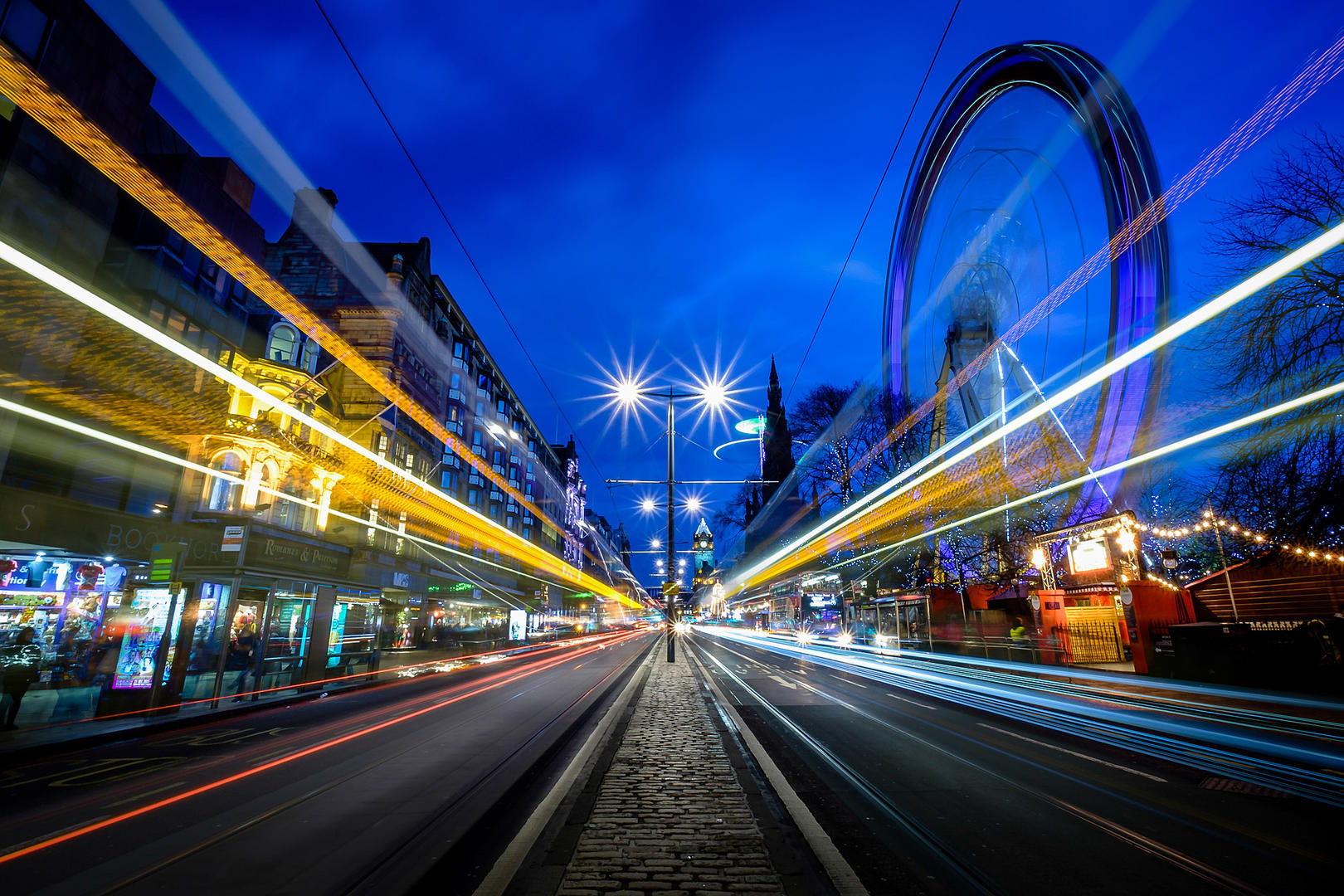The photograph is a captivating outdoor scene taken at night, employing a time-lapse technique to capture a bustling urban area illuminated with a myriad of vibrant lights. In the center of the image is a streetlight standing tall on what appears to be a small cobblestone island dividing two sides of traffic, each with three lanes. Instead of visible cars, there are mesmerizing streaks of light in red, blue, and yellow caused by the moving vehicles, hinting at possibly double-decker buses, reminiscent of London.

To the right of the photograph, an amusement park is visible, marked by a prominent ferris wheel. The stationary parts of the ferris wheel are distinguished, while the moving sections create a dazzling circle of streaks in black, blue, and green. Adjacent to the amusement park are brightly lit storefronts and a gated entrance.

On the left side, the scene transitions to a collection of illuminated buildings and shops, contributing to the overall lively atmosphere. The blue sky adds a contrasting serene backdrop to the vibrant street below. A path, likely made of cobblestones, leads from the center of the foreground of the photo toward the streetlight, enhancing the depth of the picture. Scattered around the image are various colored lights—white, orange, yellow, pale pinkish, and light blue—adding to the dynamic and vibrant nature of this picturesque cityscape. 

Overall, the photograph beautifully captures the energy and movement of an urban night, with a perfect blend of static architectural details and the flowing dynamism of a city in motion.